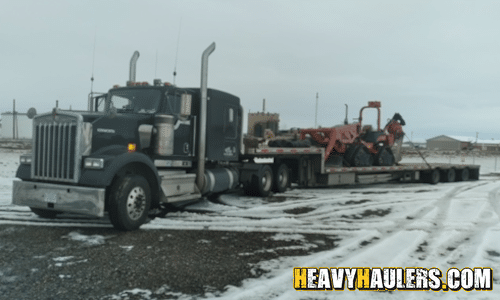In this winter landscape, a dark gray or very dark blue American semi-truck, adorned with chrome accents and boasting two large exhaust pipes on either side, is captured in motion or possibly parked on a gravel and dirt path blanketed with snow. The 18-wheeler, seen from the driver’s side, pulls an open flatbed trailer carrying a large, heavy orange construction tractor. This tractor, equipped with tracks rather than wheels and featuring a substantial front scoop reminiscent of a bobcat, appears securely fastened and positioned centrally on the trailer, which is equipped with multiple wheels to ensure proper weight distribution. In this industrial environment, with a gray, hazy overcast sky above, a building with a snowy roof is visible in the background. The image includes bold text in the bottom right corner reading "heavyhaulers.com," with yellow H's and the remaining letters in white.